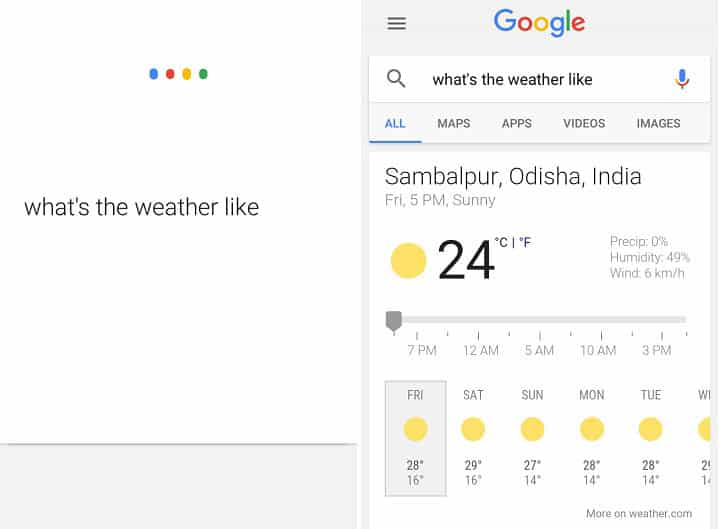A vertical screenshot captures a Google search query about the weather, framed within a typical mobile interface. The white background of the webpage highlights various colorful elements throughout the image. On the left-hand side, four circles in Google's signature colors—blue, red, yellow, and green—add a touch of vibrancy. The top of the screen displays the Google logo, accompanied by three horizontal bars indicating additional options. The search bar, complete with a magnifying glass and a microphone icon, poses the query, "What's the weather like?" in black text.

Directly below, the search results prioritize the "All" tab, which is highlighted in blue among other options like Maps, Apps, Videos, and Images. The weather information for Salman, Balpur, Odisha, India, at Friday 5 p.m., is detailed: sunny weather iconified by a yellow sun, 24°C, 0% precipitation, 49% humidity, and 6 kilometers per hour wind speed. Beneath this, forecasts for different times and days are listed, providing a comprehensive weather outlook.

At the image's bottom, a black or gray rectangular box serves as a footer, demarcating the end of the content. The overall composition of the screenshot is clean and straightforward, resembling the typical layout users expect from a Google search on a smartphone.